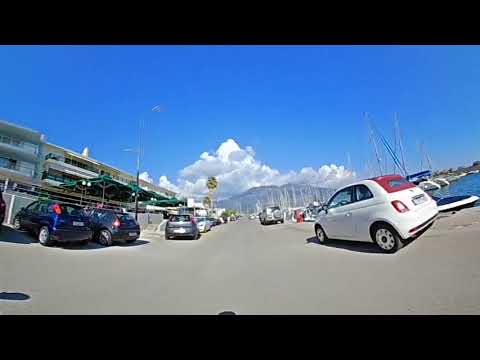This image portrays a bustling parking lot by a harbor under a bright, sunny sky. The scene, set against a large mountain with fluffy white cumulus clouds and a crisp blue sky, includes various cars parked along an inclined road. On the left side of the image, dark blue and black compact cars, as well as a silver SUV, are neatly lined up in front of a beige building with blue trim and green umbrellas. The right side features a white compact car with red taillights parked alongside a red hatchback and another vehicle. In the background, a small body of water dotted with boats adds to the harbor atmosphere. While there are no visible pedestrians in the immediate foreground, distant figures can be faintly seen. This scene captures a tranquil day near what could be a beach, complete with the necessary amenities for visitors.